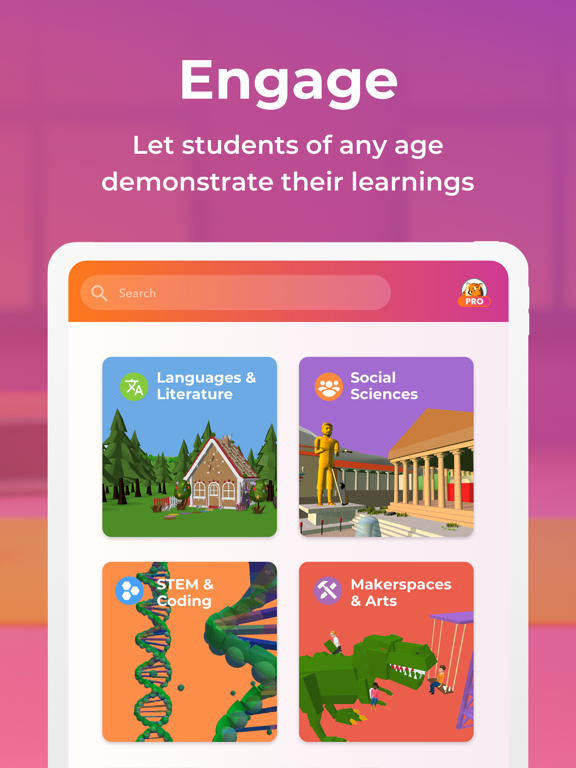In this image, we observe a vibrant page dominated by a purple and pink color theme. The central text proclaims, "Engage: Let students of any age demonstrate their learning." Beneath this statement is a search bar, accompanied by a "Pro" button positioned on its right. 

The page is divided into four distinct sections, each denoted by an emblem illustrating different learning categories:
1. **Languages and Literature** - Represented by an image of a quaint house nestled in the woods.
2. **Social Sciences** - Illustrated with a picture reminiscent of ancient Italian or Greek architecture, highlighted by classical buildings.
3. **STEM and Coding** - Featuring a vivid green DNA helix.
4. **Makerspaces and Arts** - Showcased by a playful depiction of a large Lego-like dinosaur with a child swinging from it, emphasizing a sense of creative freedom.

This layout encourages users to select from these diverse educational pathways, each designed to engage students in demonstrating their learning through various themes and activities.